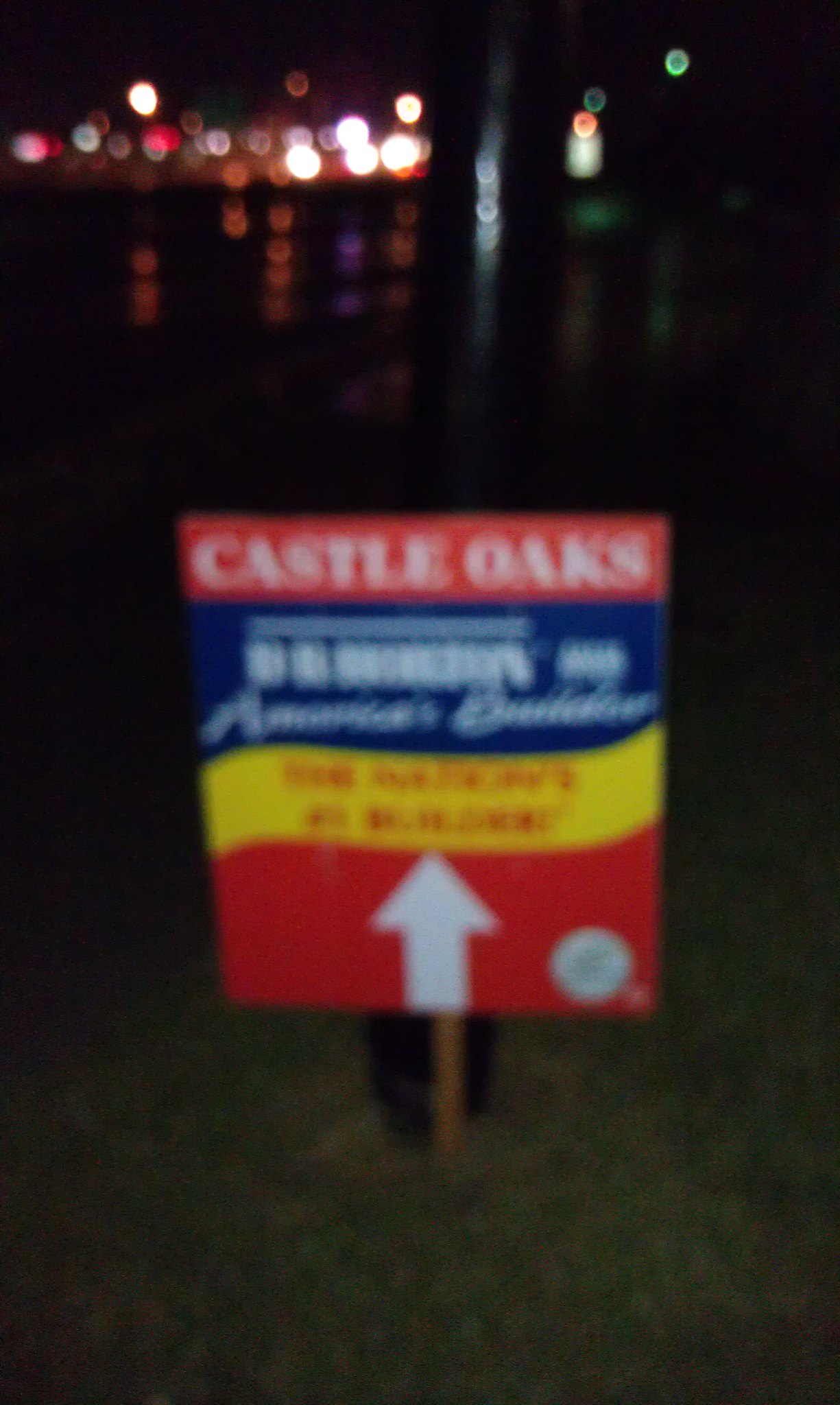In this blurry, vertical night-time photograph, likely illuminated by automobile headlights, a slightly rectangular sign is prominently featured at the center. The sign is mounted on a brown metal pole and consists of sections colored red, blue, yellow, and red from top to bottom. In the uppermost red section, white letters spell out "Castle Oaks." Below this, the blue segment contains additional, unspecified text. The yellow section also features writing, including a phone number. The lower red section of the sign is marked by a white circle in the bottom right corner and a large white arrow in the center, pointing upwards towards the phone number and other text above. In the distant background, lights from buildings and cars are faintly visible, suggesting an urban setting. The wet, rainy conditions are evidenced by the shiny reflection on the surface, adding to the overall blurred effect of the image.